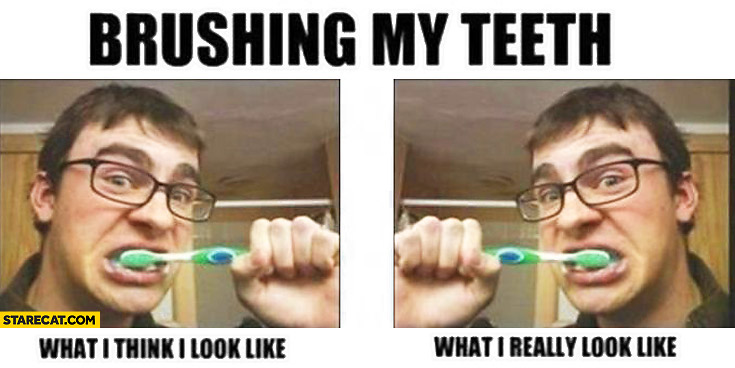The meme features a young white man, probably in his early-to-mid 20s, with brown hair and bushy eyebrows, wearing dark brown or black glasses, brushing his teeth. The image is split into two side-by-side identical photos on a white background. The black, bold caption at the top reads "BRUSHING MY TEETH" in all capital letters. Under the left photo, a caption says "WHAT I THINK I LOOK LIKE," and under the right photo, it says "WHAT I REALLY LOOK LIKE." 

In both photos, the man is facing the camera while brushing his teeth with a toothbrush that is primarily white with bright green and blue accents. He is wearing a black shirt. The left image shows the man slightly angled to the left, while the right image is a mirror version with the man slightly angled to the right.

Behind him, the visible background includes brown cabinetry, likely indicating a bathroom setting, and a ceiling, as well as what appears to be a rod for a shower curtain. The overall scene is set indoors, probably in his home.